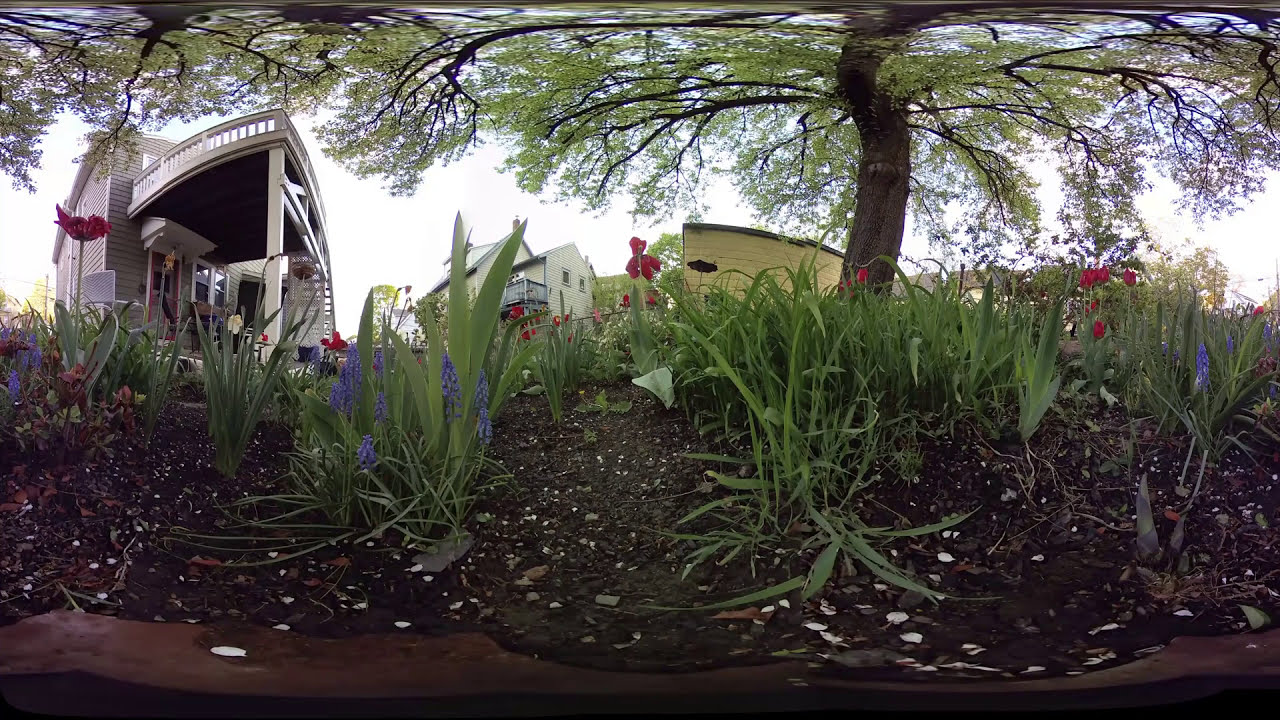This photo portrays a detailed scene of a lush yard and an adjacent multi-storied white house situated on a small hill. The image is horizontally rectangular and primarily dominated by dark, fertile soil speckled with white flecks. Emerging from the soil are vibrant blades of grass, and blooming amongst them are delicate red and purple flowers, seemingly lavender.

In the midground, standing tall and shading part of the yard, are two large trees with abundant green leaves. To the left, a distinctive white porch forms a V-shape and is supported by a white column. This porch is part of a gray, multi-storied house with a notably pink door and a second-floor balcony. The porch on the first floor features a chair and hanging planters, adding to the picturesque charm. Adjacent to this structure is another house, painted a pale yellow with a blue balcony, followed by a light green or possibly yellow building, visible as a small sliver.

Adding to the serene atmosphere, the sky stretches beautifully blue without a hint of clouds, providing a perfect backdrop for this quaint and vibrant scene.